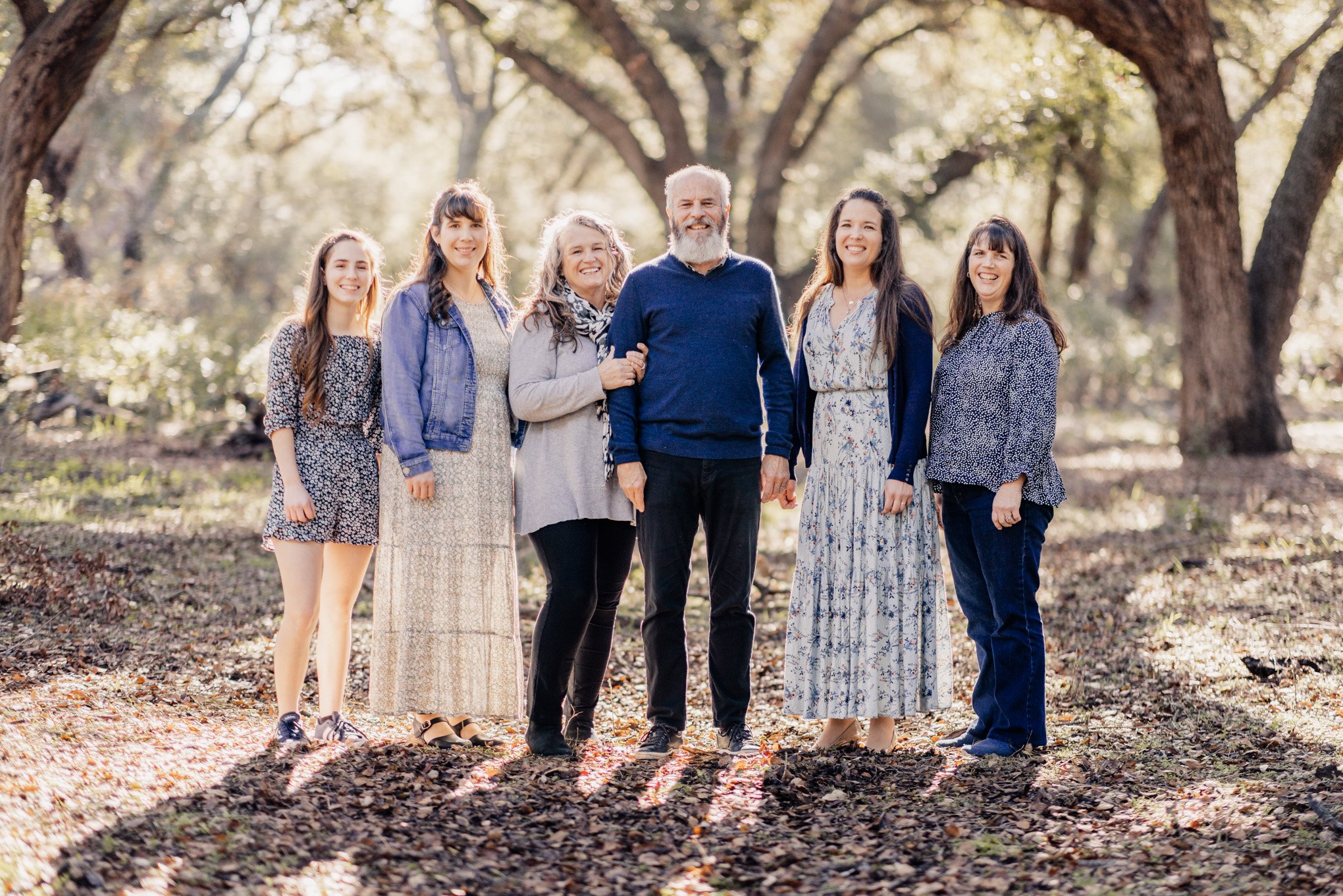In this high-quality, landscape-oriented photograph, six people stand together amidst a forested backdrop, where blurry trees can be seen along with a forest floor covered in dirt and dead leaves. At the center of the image are an elderly Caucasian couple: the woman, wearing a gray shirt paired with a scarf and black pants, has long gray hair, while the man next to her sports a long-sleeve blue shirt, black pants, white hair, and a beard. Flanking them are their likely daughters—two women to the left in their 20s with long brown hair, and two women to the right, probably in their 30s or 40s, also with long brown hair. All six individuals are smiling and looking towards the camera, illuminated by the natural daytime light that enhances the photo's clarity and detailed depiction of this loving family moment.